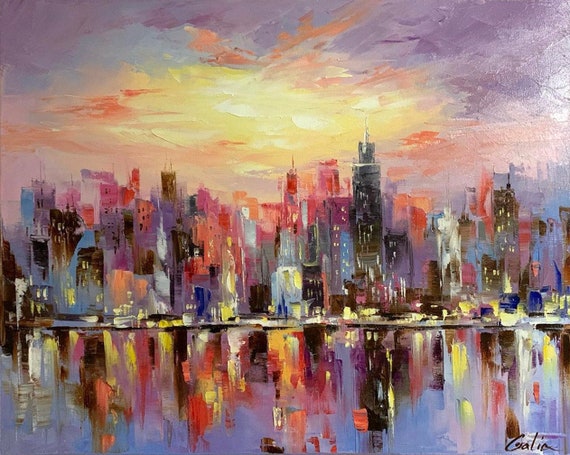This painting depicts a cityscape, reminiscent of New York City, positioned right on the water's edge. The scene showcases a variety of tall buildings in different sizes, with their reflections vividly mirrored in the blue water below, establishing a captivating and somewhat abstract aesthetic. The sky above is painted in muted shades of purple, blue, yellow, and orange, providing a soft yet vibrant backdrop. 

Some of the buildings in the background are illuminated with orange hues, creating a warm contrast, while the visible lights in the windows add yellow accents throughout the composition. Darker buildings dominate the foreground, with blue tones prominent in the scene. The artist's signature, possibly "G-A-L-I-A," can be discerned in black in the lower right-hand corner on the blue water. The overall impression of the artwork is both blurry and abstract, blending colors and shapes to evoke the dynamic essence of a city by the water.